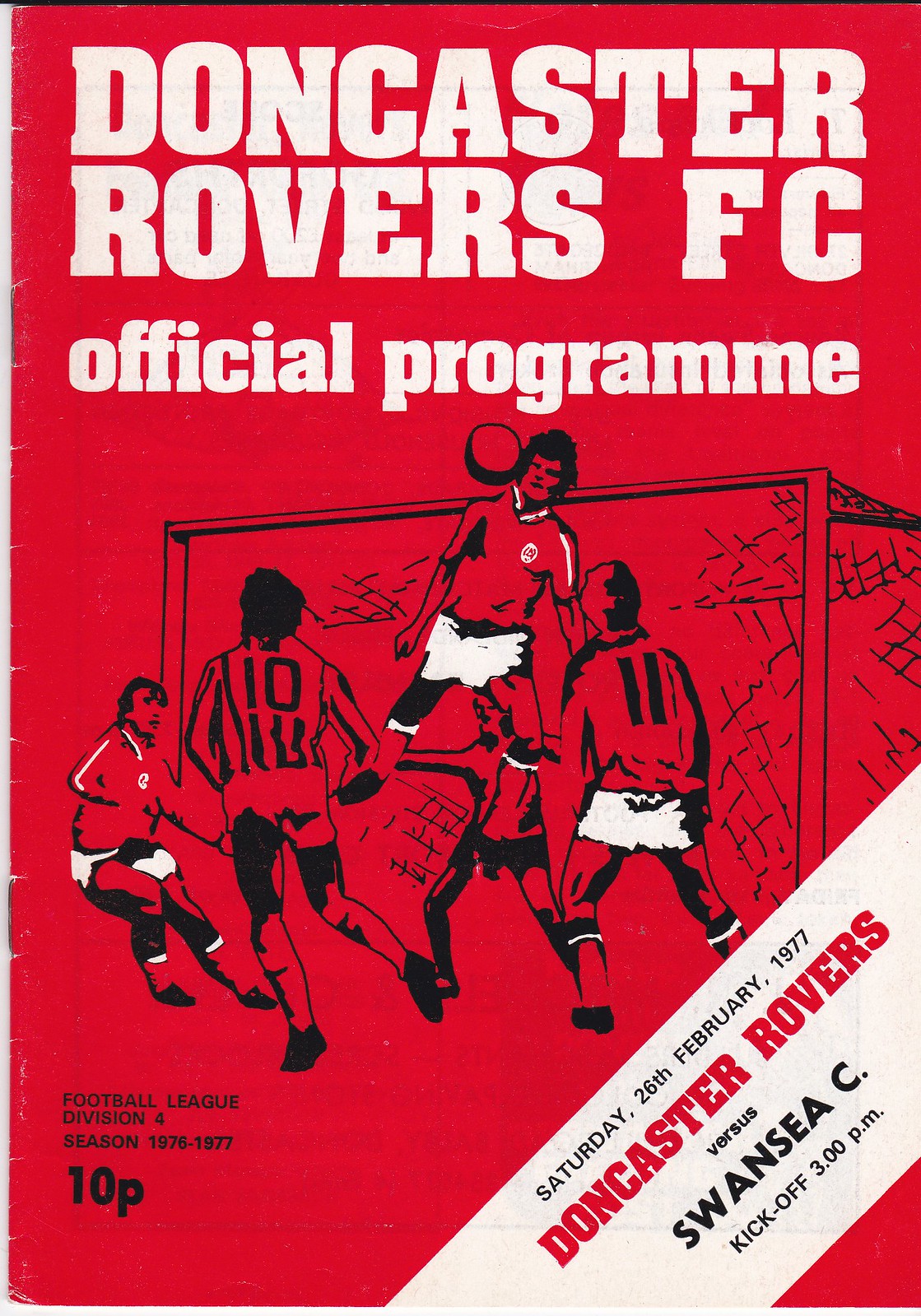The image shows a red, rectangular, portrait-oriented front cover of a football match program or booklet. The top of the cover features the white text "Doncaster Rovers FC Official Program." Below this, a black outline of a goalpost net and an action-packed sketch in black and white depict a football player leaping into the air with the ball just in front of his face, surrounded by four players wearing yellow shorts, with numbers such as 10 and 11 on their backs. At the bottom left, black text reads "Football League Division Four, season 1976-1977 10b." A white diagonal banner runs down the bottom right, displaying in black text "Saturday, 26 February 1977," followed by "Doncaster Rovers versus" in red and "Swansea C" in bold black, with a kickoff time of 3 p.m. The dynamic cover reflects the competitive spirit of the match.